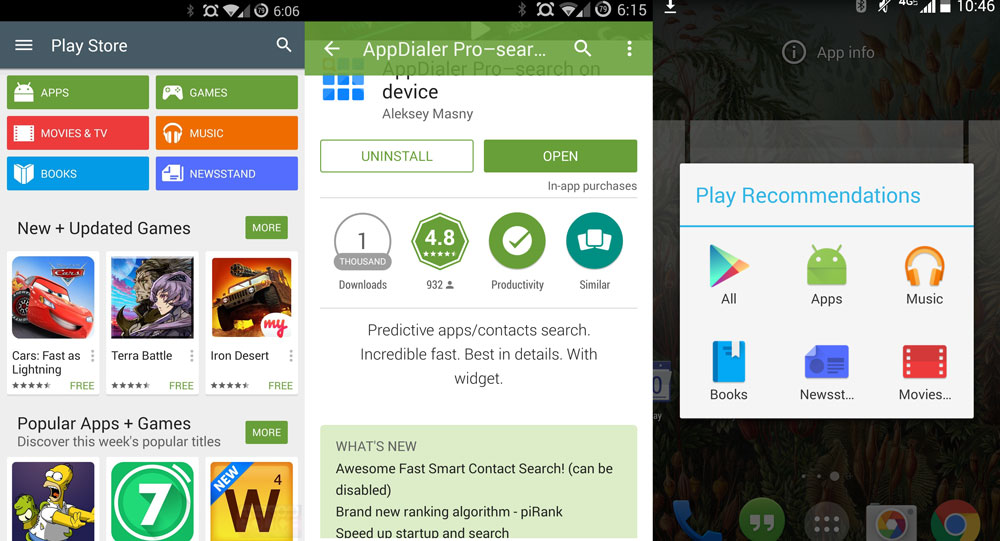This image consists of three different screenshots from the Google Play Store, arranged side by side to appear almost as a single page. A closer look, however, reveals that each is a distinct screenshot, identifiable by the black top border featuring typical smartphone status icons such as the time, Wi-Fi connection, and battery indicator.

The first screenshot on the left showcases the Play Store interface. Directly below the black border is a dark gray header with the text "Play Store" in white. Beneath this header are several colored rectangular tabs: green for "Apps," green for "Games," red for "Movies & TV," orange for "Music," sky blue for "Books," and a medium to light blue for "Newsstand." Following these tabs is a section labeled "New and Updated Games," displaying thumbnails of six different games arranged in two rows of three.

The middle screenshot features the page for a specific app, identified as "App Dialer Pro." Below the typical black border, the header is an olive green with the title "App Dialer Pro - Search" partially visible. This indicates that the user is viewing detailed information about this particular app.

The rightmost screenshot presents a pop-up window against a black background. The pop-up, with a white background and blue headline, is titled "Play Recommendations." It displays categories such as "All," "Apps," "Music," "Books," "Newsstand," and "Movies," each accompanied by corresponding icons.

Together, these screenshots provide a comprehensive overview of different facets of the Google Play Store, from browsing categories to viewing individual app details and receiving personalized recommendations.